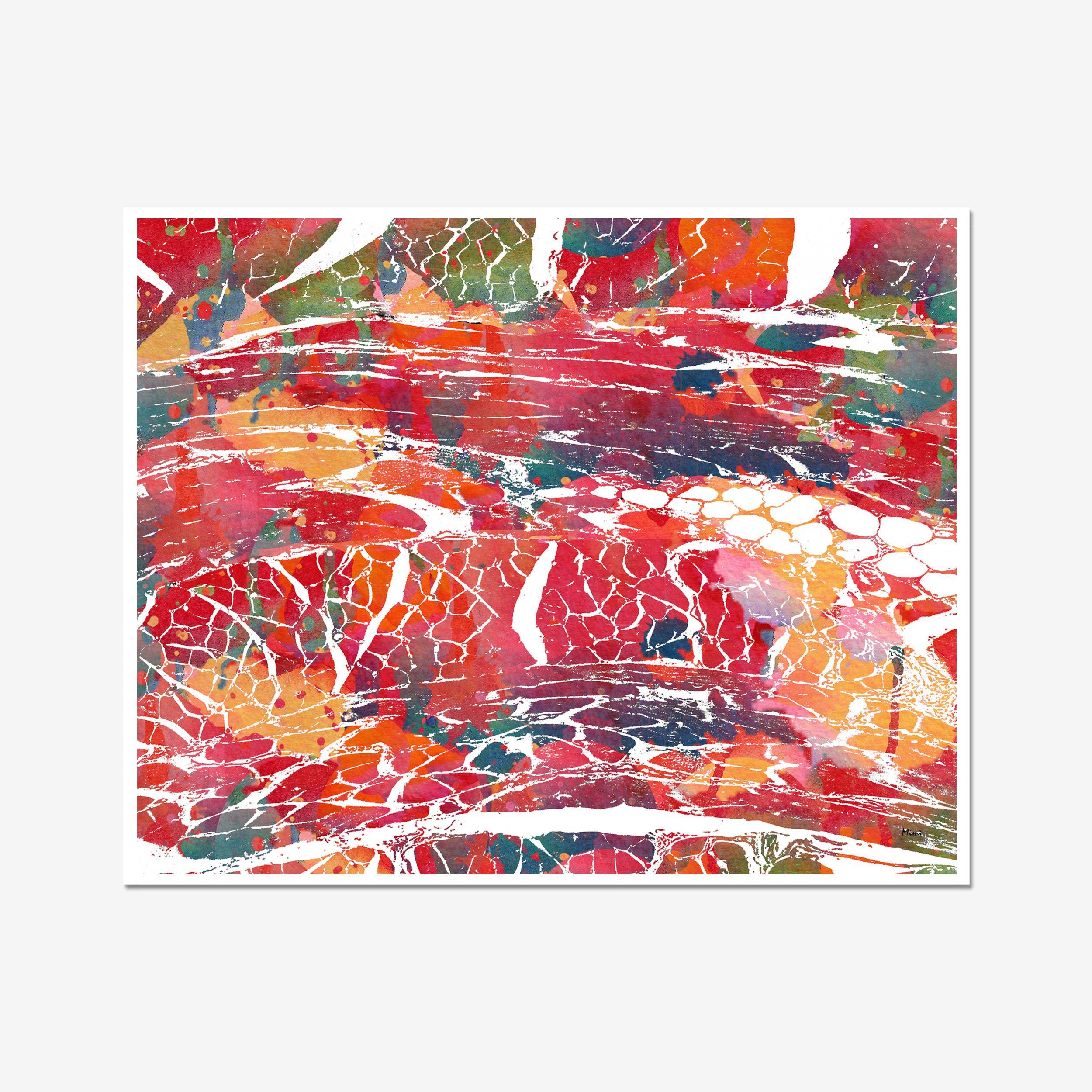The image depicts an intricate, abstract painting displayed on a grey wall. The canvas is vibrant and uses a predominant palette of red, orange, green, and blue. The abstract composition includes various shapes reminiscent of cobblestones or a watery surface, appearing both fragmented and interconnected. White lines and dots are scattered throughout, adding to the complexity and dynamic feel of the artwork. The top left corner is primarily red, blending into green and white, transitioning to red and blue in the center, and finally into orange in the top right corner. The painting captures an underwater-like scene with decorative, undefined shapes that mix and overlap, giving it a three-dimensional, almost popping-out effect. The image evokes a sense of movement and depth, making it an intriguing and captivating piece to observe.